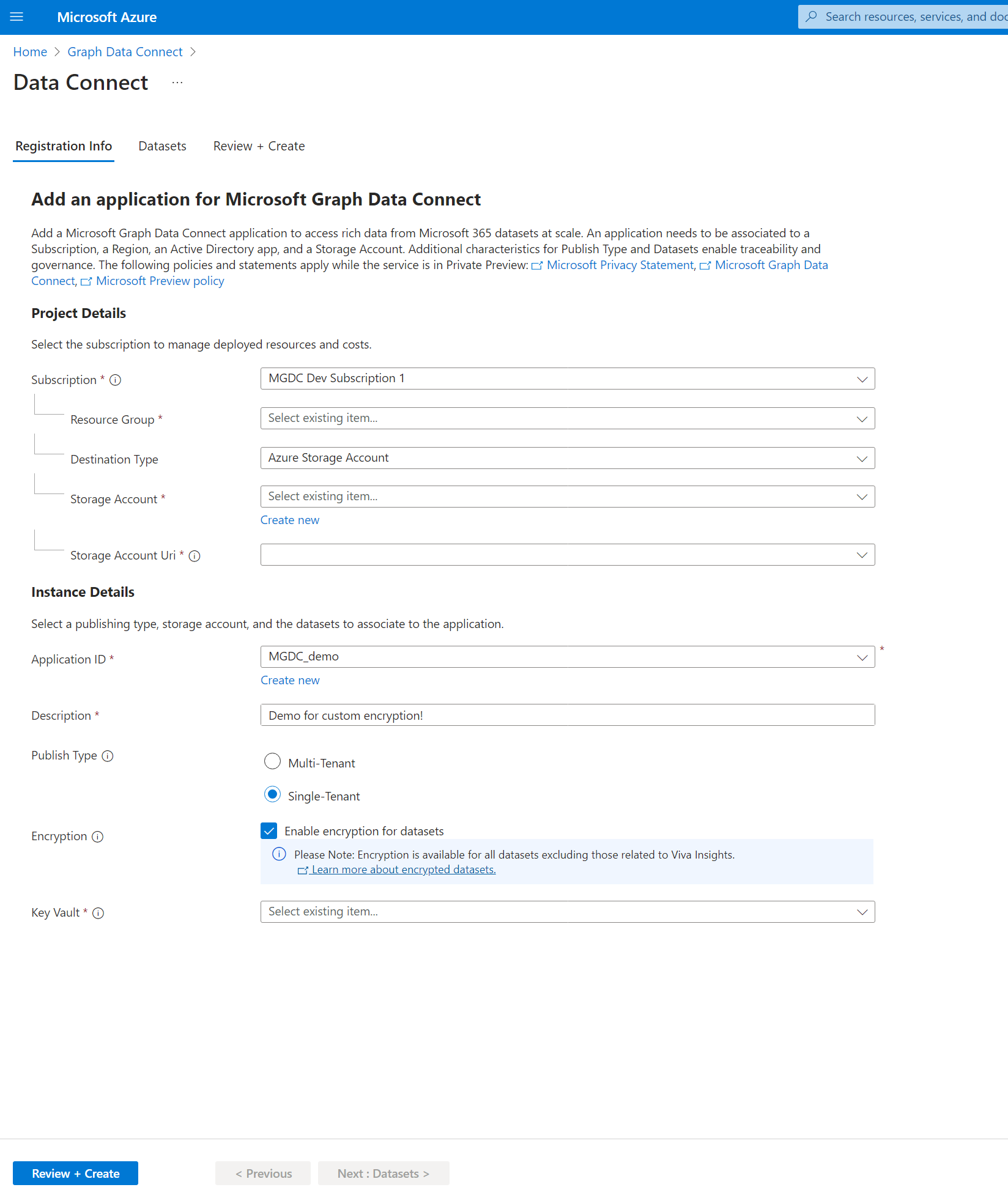This image is a screenshot from a programming or website diagnosis page on the Microsoft Azure platform. The photo is portrait-oriented, significantly taller than it is wide. At the top, there's a blue horizontal header featuring a slightly obscured icon and white text that reads "Microsoft Azure," accompanied by a grey search box on the right side.

Below the blue header, the background shifts to white, displaying a breadcrumb navigation with blue links indicating the path: Home > Graph Data Connect. Under this, a black header labeled "Data Connect" is visible, followed by several selectable options: Registration Info, an unreadable option, and Review and Create. The "Registration Info" option is highlighted in bold with a blue underline, indicating it is currently selected.

The main content area starts with the title "Add an Application for Microsoft Graph Data Connect" and includes a paragraph of explanatory text. Below this, there's a subheader titled "Project Details," which lists various terms with corresponding checkboxes and dropdown menus for specific selections to the right. Further down, there is another header labeled "Instance Details," featuring mandatory fields denoted by asterisks, each accompanied by dropdown boxes and radio buttons meant for user input.